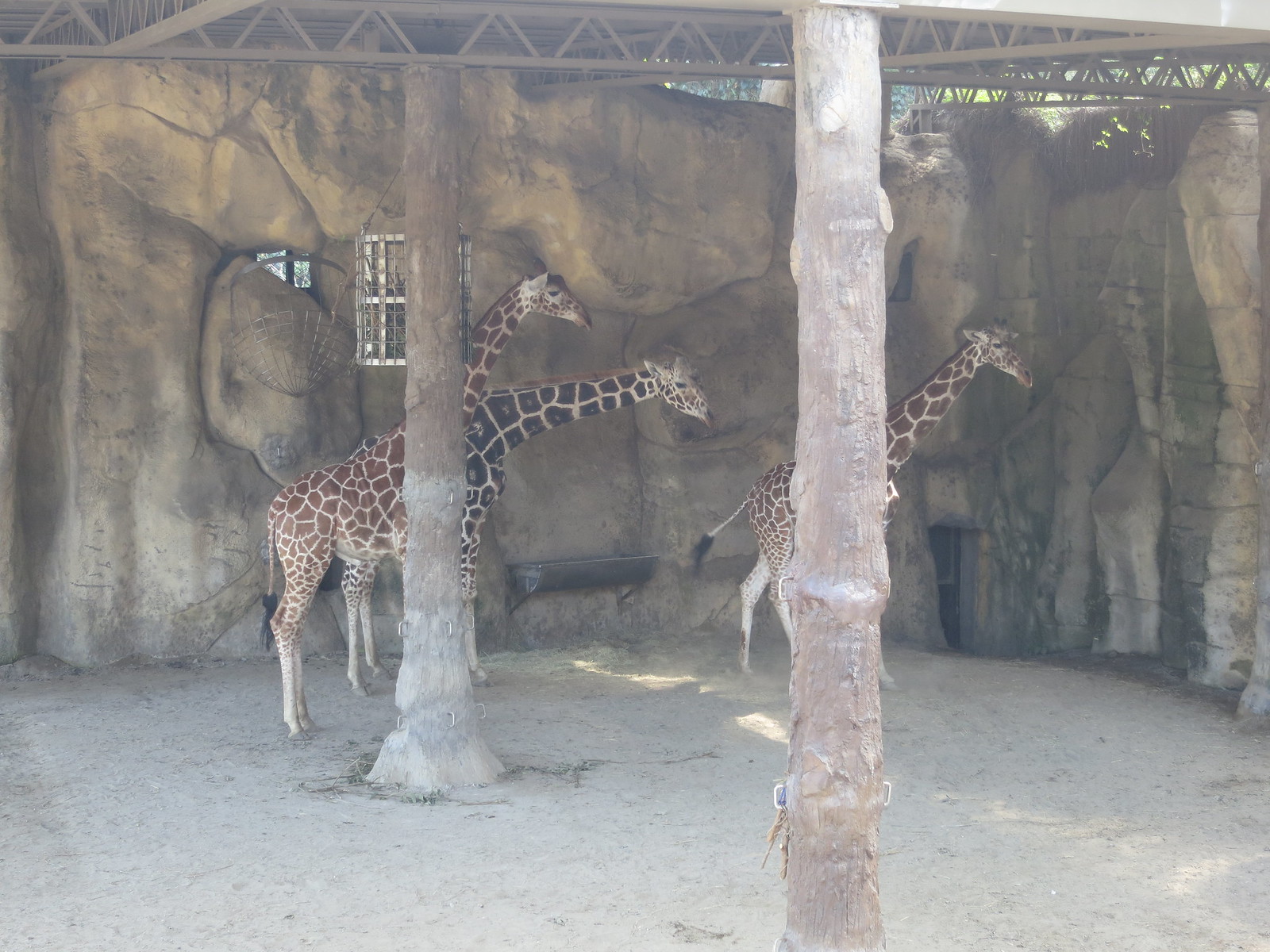This photograph captures three giraffes in a zoo enclosure, standing in an enclosed area with man-made rock walls in the background and a sandy, possibly sandy-concrete ground. Two prominent tree trunk-like pylons obstruct the view, running vertically through the image and partially covering the giraffes' bodies. The tallest pylon appears to support scaffolding adorned with a small white window at the top. The giraffes, likely adolescents due to their shorter necks and legs, exhibit a range of slightly downward neck postures. The giraffe on the right seems younger than the others. A small water trough is visible at the base of the rock wall, designed for the giraffes to drink from.